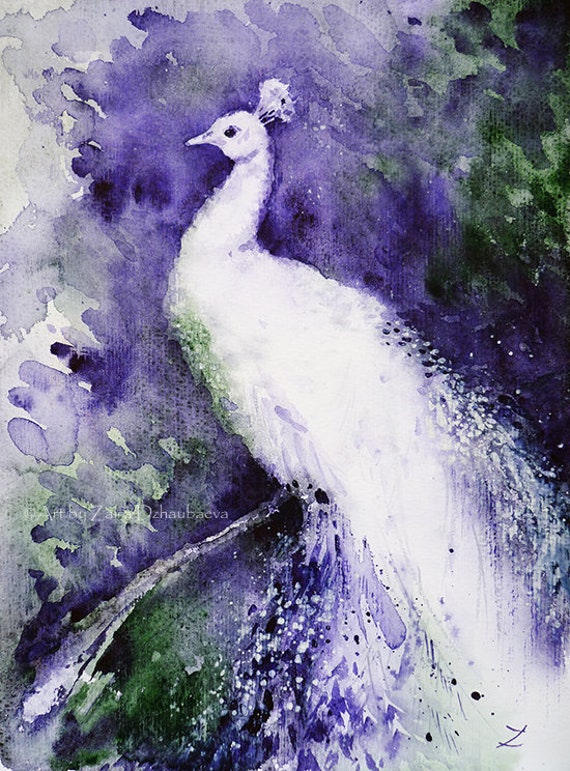This is a detailed watercolor painting featuring a stylized, artistic depiction of a peacock. Predominantly white, the peacock is rendered with delicate feathery wisps that fade toward the bottom, emphasizing the ethereal quality of its plumage. The bird is positioned centrally in the image and oriented to the left, showcasing its profile with a distinct black eye. Surrounding the peacock, various intense shades of blue are applied in splotches, outlining and defining the bird's form. Subtle green highlights enhance the composition, appearing notably in the upper right-hand and lower left-hand corners to add depth and contrast to the primarily bluish background. There are also hints of purple interspersed throughout the image, particularly in the left part of the background, which transitions from dark to lighter shades. Additionally, a small, barely discernible white text at the bottom left, starting with a 'Z' and 'D,' marks the artist's signature. Overall, the painting harmoniously blends colors to produce a relaxed yet striking visual experience.